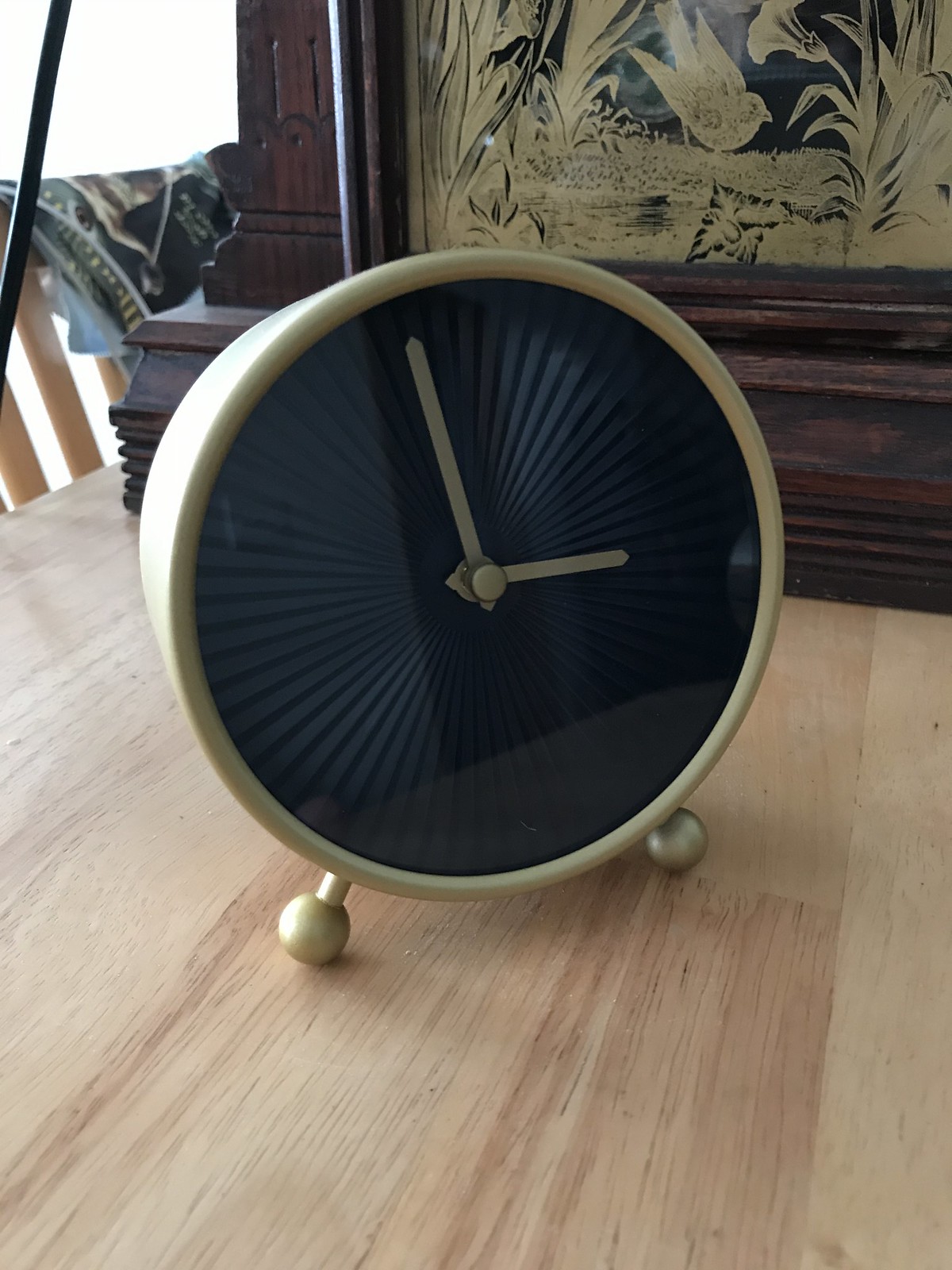This color photograph captures an indoor scene centered around a small, intricately designed desk clock placed on a beige wooden surface, likely a table. The clock, with its brushed bronze frame and ball-shaped feet, stands elegantly, featuring a black, vent-like face without any numbers, and bronze hands indicating the time to be almost 3 o’clock. Behind the clock is a dark wooden structure adorned with a painting depicting yellow birds and flowers against a black background. A green and brown fabric, possibly a shirt, is draped over a nearby railing, partially visible in the background.